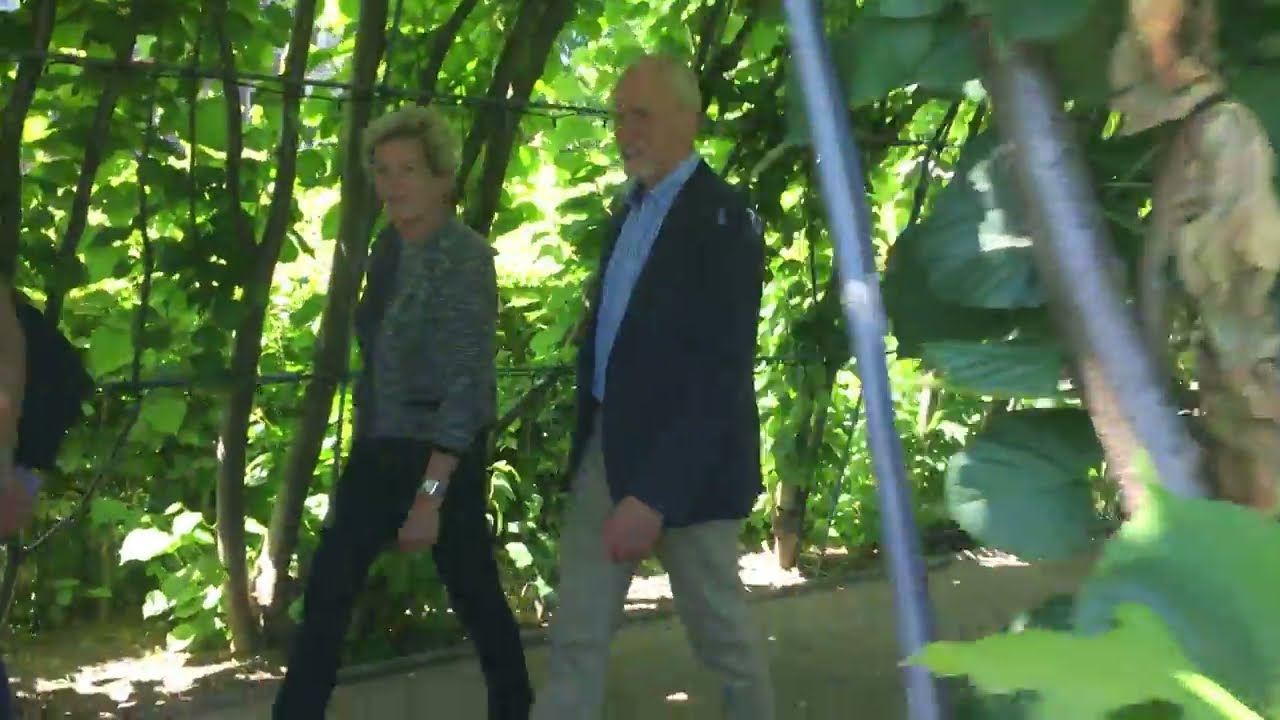The image captures the serene and meticulously designed Kensington Gardens, showcasing one of its elegant rectangular ponds. Encircled by a gray stone tile walking path, the garden is lush and vibrant with greenery. Verdant trees, green bushes, and immaculately manicured lawns add richness to the scene, visually striking against the backdrop of a clear, blue sky. White flowers are interspersed throughout the garden, adding a touch of purity amidst the green. 

The pond itself is adorned with various types of plant pots and planters, some placed in wooden crates and round pots along the perimeter, while three large brick planter boxes appear to float on the water's surface, spray misting water gracefully from their tops. This blend of green foliage and white blooms provides a calming sight. The pond is accessible via stone staircases from multiple directions. An old red brick wall partially encloses the area, lending a historic charm to this beautifully landscaped and idyllic setting.